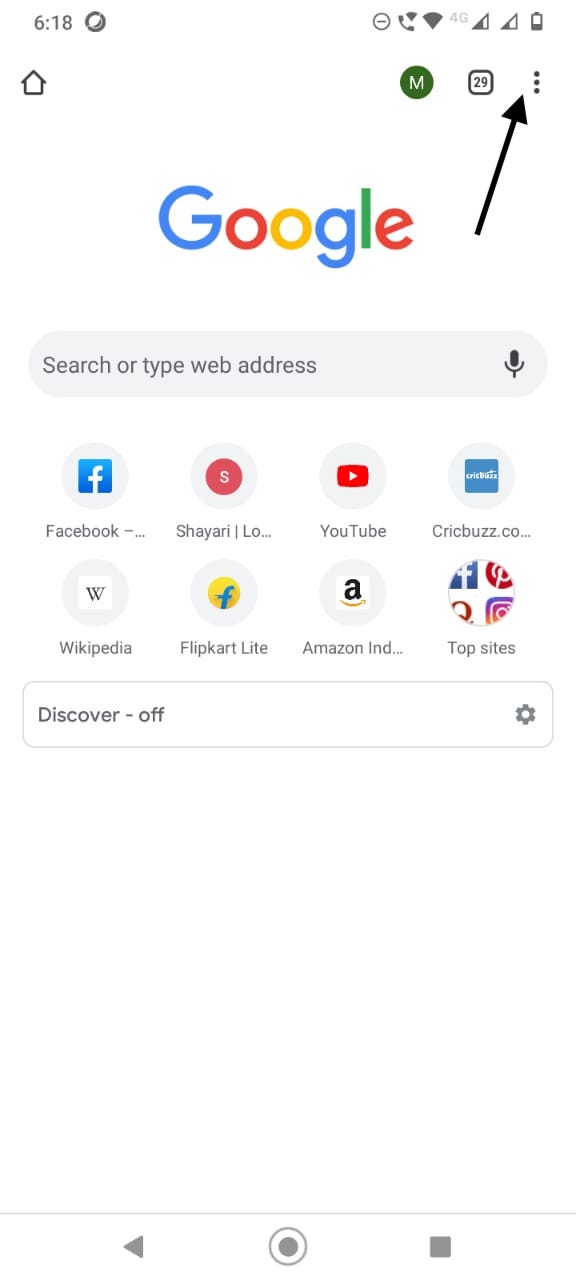The image depicts a smartphone screen displaying the Google app. The time shown on the phone is 6:18. In the top right corner, there's an indication that the user's profile name starts with the letter "M," and they have 25 messages or notifications. The main feature of the screen is the Google search bar situated prominently in the center, with options to either type a web address or initiate a voice search.

Below the search bar, there are several icons for quick access to popular sites, including Facebook, YouTube, Wikipedia, Flipkart Lite, Amazon, and a section labeled "Top Sites" and "Discover." These appear as clickable shortcuts. Further down the screen, it seems there is a drop-down menu or configuration option.

At the very bottom of the screen, the phone's navigation buttons are visible, providing the user with the means to exit the current app or switch to another application.